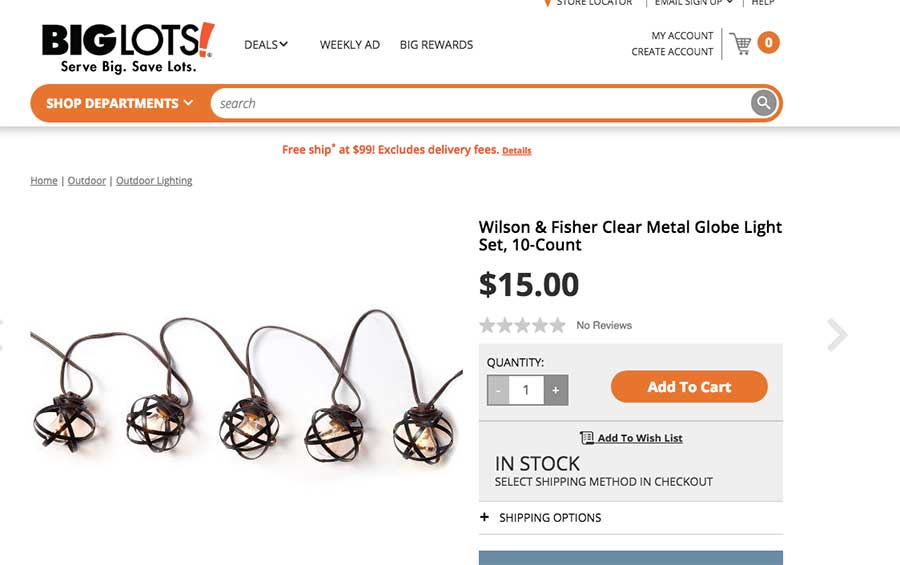In this vibrant and detailed promotional image from the Big Lots website, the banner prominently announces the store's slogan, "Serve big, save lots," with the word "big" in a bold font and an eye-catching large orange exclamation point next to "lots." 

At the top of the image, navigation options are displayed, including "Deals," "Weekly Ad," "Big Rewards," "My Account," and "Create an Account." The shopping cart icon indicates there are no items currently in the cart, marked by a zero. Additionally, a notification promises "Free ship at $99," with a note that delivery fees are excluded.

Scrolling down, there's a clickable menu bar with categories such as "Home," "Outdoor," and "Outdoor Lighting." The main feature of the image is a charming set of decorative lights. These lights are beautifully crafted with twine wound around them, perfect for outdoor settings. The product is identified as the "Wilson and Fisher Clear Metal Globe Light Set," available in a 10-count set for $15. 

Further options allow users to add the item to their cart or to a wish list. The product is in stock, and shipping options are provided for customer convenience.